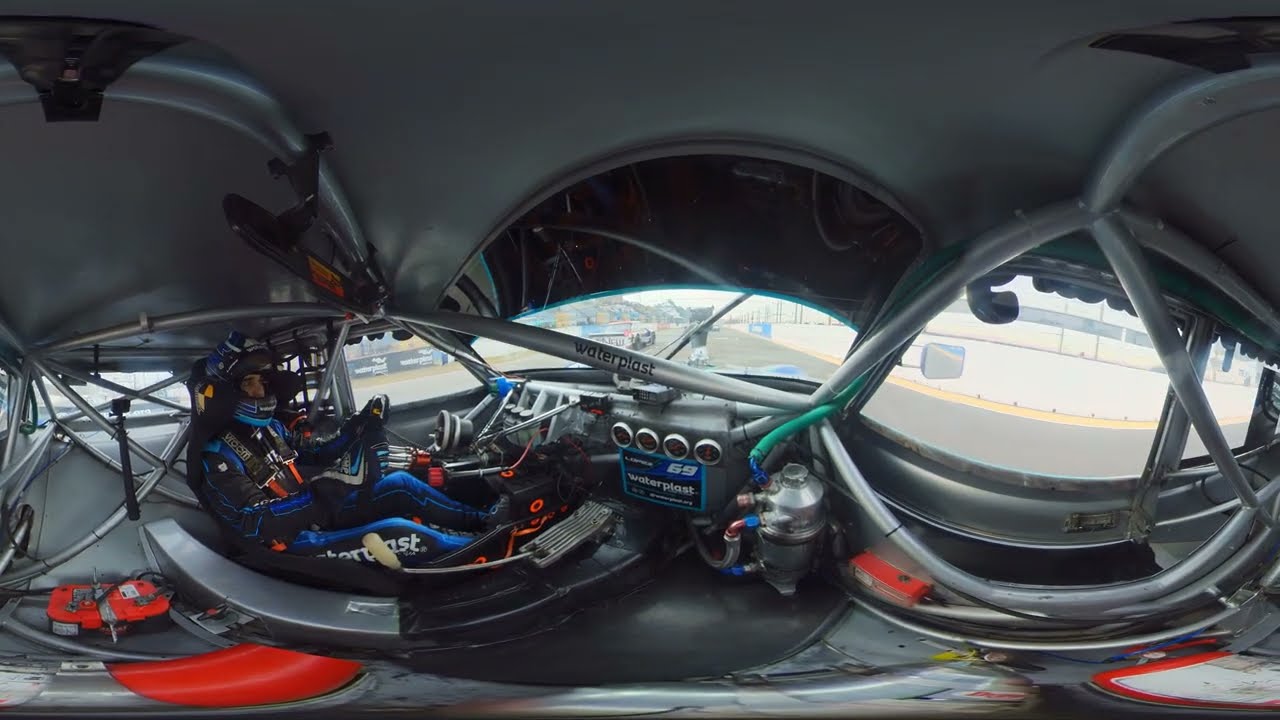The image is a 360-degree panoramic shot inside a race car on a racetrack, taken during the daytime. The driver, situated on the left side of the vehicle, is dressed in a blue, black, and white racing suit with white text along his leg and a matching helmet with the visor up, revealing his face. He is securely strapped into his seat with black shoulder straps and is holding the steering wheel firmly. Surrounding him is an intricate framework of interconnected steel bars forming a protective roll cage, along with various curved silver poles inside the vehicle. Visible in the front right of the car is a tank with tubes and black dials. A series of gauges and instruments span the dashboard area in front of the driver. Out the windows, the racetrack is visible with painted advertisements along the edges. The landscape outside includes signs on the fence bordering the track, and in the distance, another race car can be seen. The interior of the vehicle is minimalist, dominated by its exposed steel structure and basic functional elements necessary for racing.